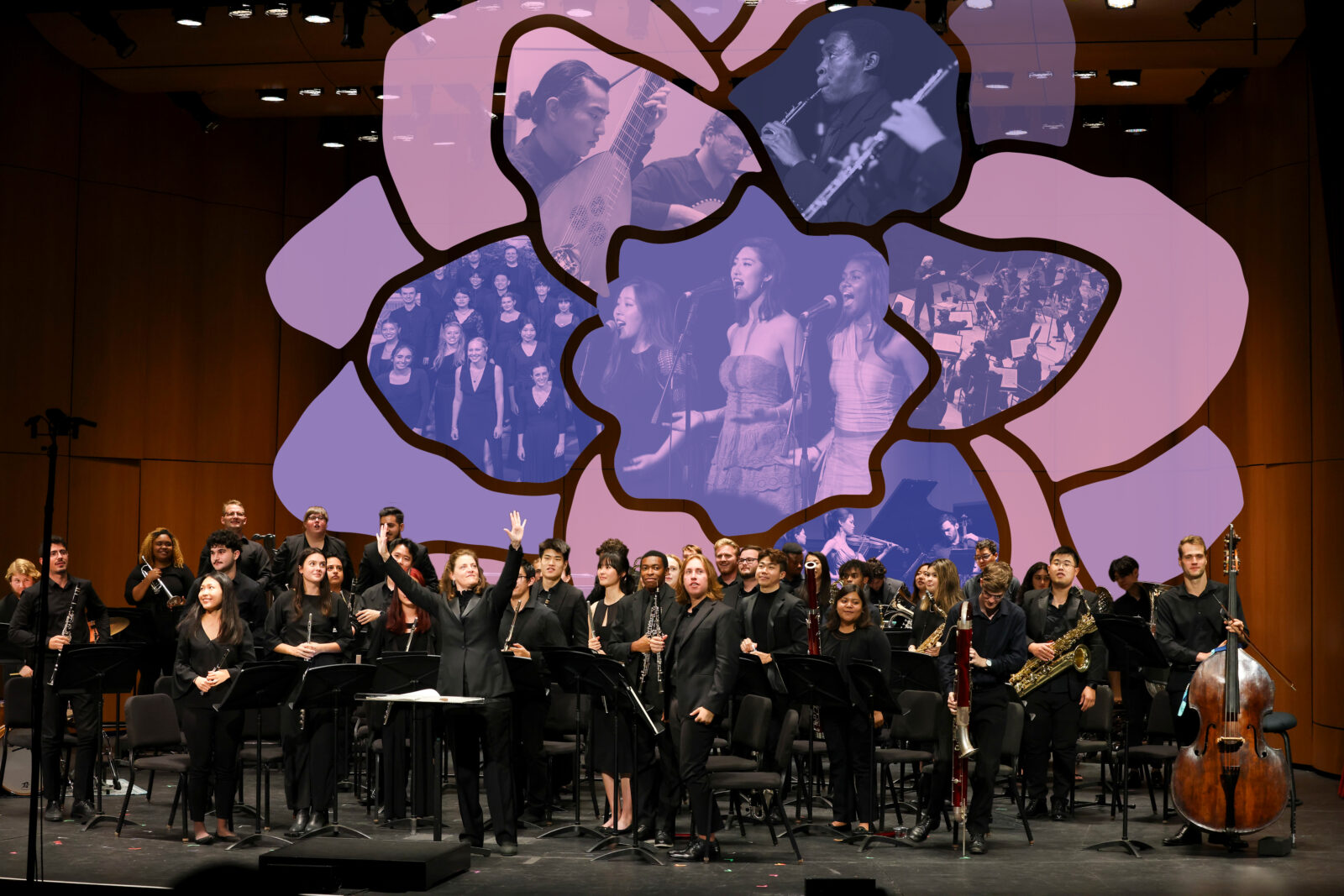The image portrays a symphony or jazz orchestra poised on a black stage, surrounded by dark wood panel walls rising from floor to ceiling. Dominating the backdrop is an artistic display of a large multi-petaled flower, with inner translucent petals featuring black-and-white images of musicians engaged in their performance. The center-most part of this floral design showcases three female singers stationed behind floor microphones. The orchestra, comprised of both male and female musicians uniformly dressed in black attire—ranging from pantsuits and dresses for the women, to black button-down shirts and pants for the men—stands resolutely, holding an array of instruments, including a brown bass prominently on the right. Completing the scene is their conductor, positioned on the left with raised arms, seemingly in a gesture of commendation directed at the ensemble. Behind each musician are slimline black chairs, further accentuating the structured arrangement of this harmonious gathering.